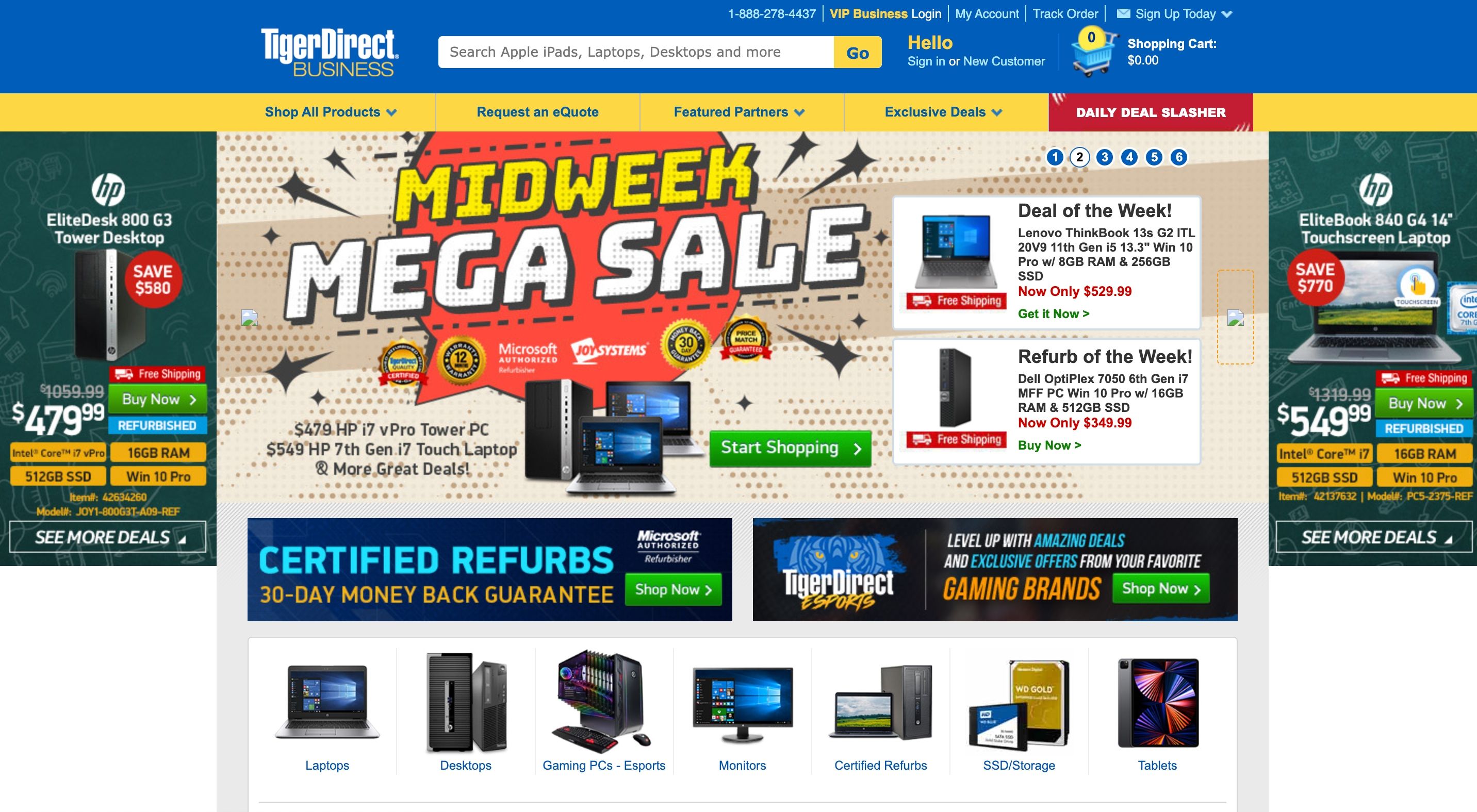This image is a screenshot from the TigerDirect business website. At the very top of the webpage, a blue navigation bar spans horizontally from left to right. This blue bar contains several elements: a search bar, a phone number, a VIP business login link, a 'My Account' option, a 'Track Order' option, and a 'Sign Up Today' option. Additionally, there is a shopping cart icon and a greeting message that says "Hello, Sign In or New Customer."

Directly beneath the blue bar is a yellow horizontal menu bar, also stretching from left to right. This yellow bar features options such as 'Shop All Products,' 'Request a Quote,' 'Feature Partners,' and 'Exclusive Deals.' Highlighted in red within this bar, the words "Deal, Daily Deal Slasher" draw attention.

Below the yellow bar, the main window of the website showcases a promotional banner for the "Midweek Mega Sale." This section includes images of computers and laptops, and prominently features a green button with white text that reads "Start Shopping."